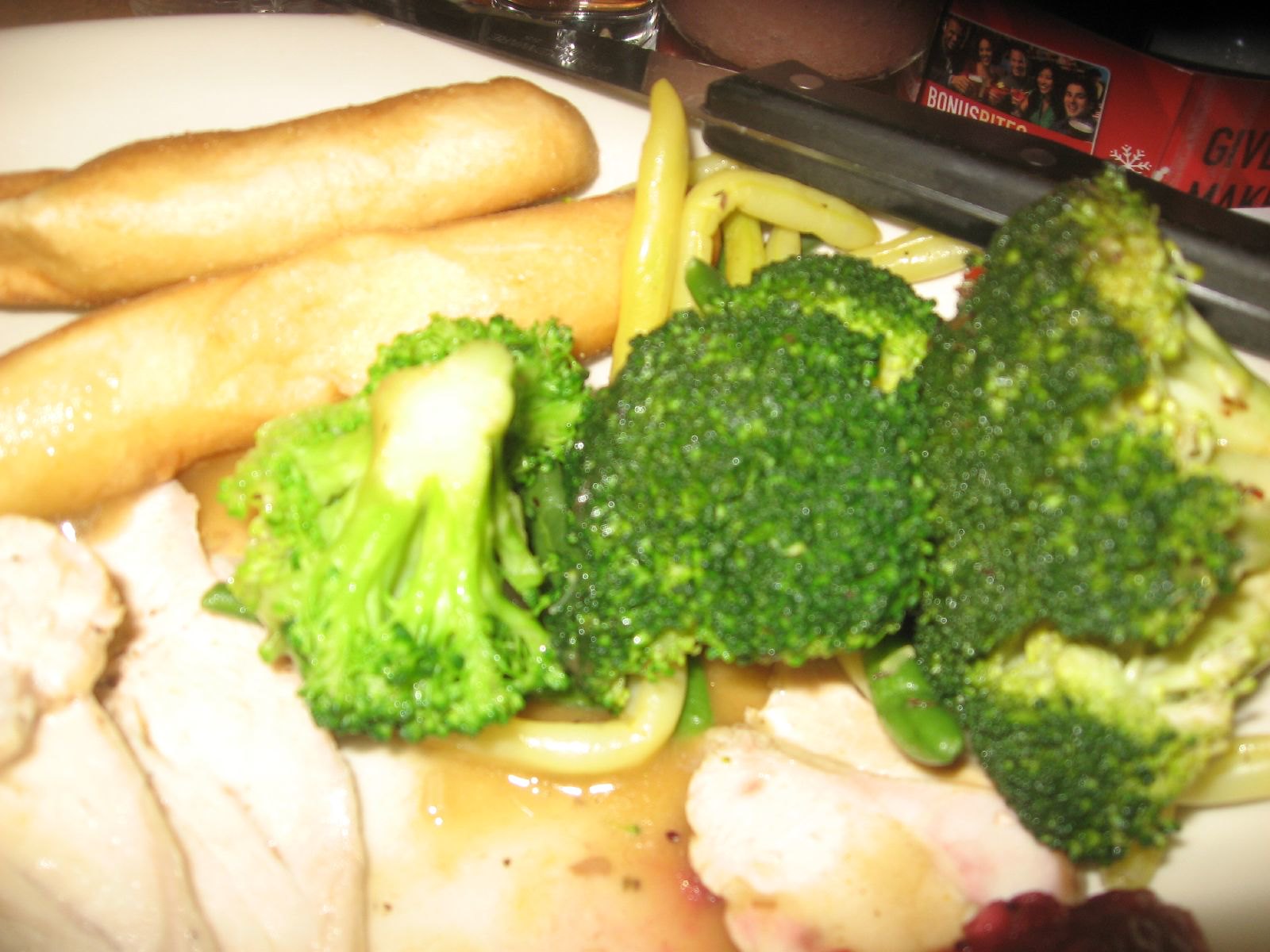This overexposed and poorly focused close-up photograph depicts a dinner plate with an assortment of foods. The left side of the image is overexposed, resulting in some areas lacking detail. At the center, several broccoli florets with bright green stems and darker green tips extend to the right. Resting on mashed potatoes, the broccoli is partially surrounded by yellow and green string beans and a puddle of what appears to be gravy. In the lower right-hand corner, a small splotch of dark red material suggests the presence of jellied cranberry sauce. Toward the back left, two rounded brown oblongs, likely spring rolls or breadsticks, are visible, along with more light lime green vegetables. Additionally, to the lower left, there are two slices of white meat poultry, possibly turkey or chicken. A knife with a black handle extends from the back rim of the plate, with its stainless steel blade reaching off the screen. The overall composition suggests a haphazardly arranged meal on a large plate or tray.